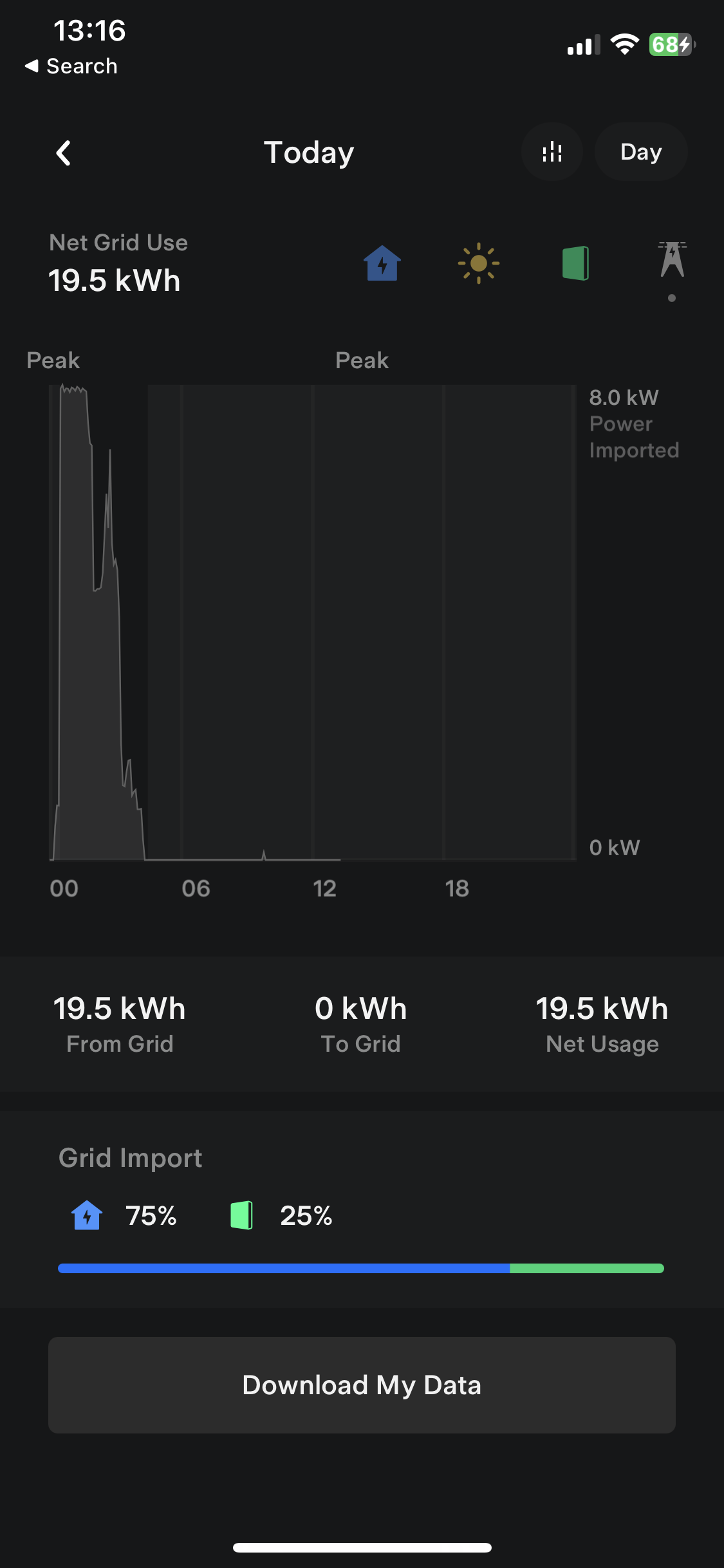This image captures the screen of someone's cell phone at 13:16 (1:16 PM). The top of the screen displays indicators for cellular signal strength, Wi-Fi connectivity, and battery charge at 68%. The date reads "Today."

Below the top indicators, the main display shows an energy usage dashboard. The dashboard features a bar graph indicating net grid usage of 19.5 kWh. The graph has labeled intervals at the bottom, reading 0, 6, 12, 18 and 24 hours, and power measurements on the right side ranging from 0 to 0.8 kW. At the top right and bottom right, "0.8 kW" is labeled for power imported.

The graph line starts on the left at 0.0 and rises sharply to a peak, then gradually declines before reaching a flat line around hour 6. Below the graph, it states "19.5 kWh from grid," along with the net usage breakdown: "75% import from house" and "25%."

Icons accompany these statistics: a blue house representing the 75% import from house and a green rectangle, possibly representing the remaining 25%.

At the bottom of the screen, there is a button labeled "Download My Data."

Overall, the display provides a detailed overview of the user's energy consumption, import stats, and the option to download data for further analysis.